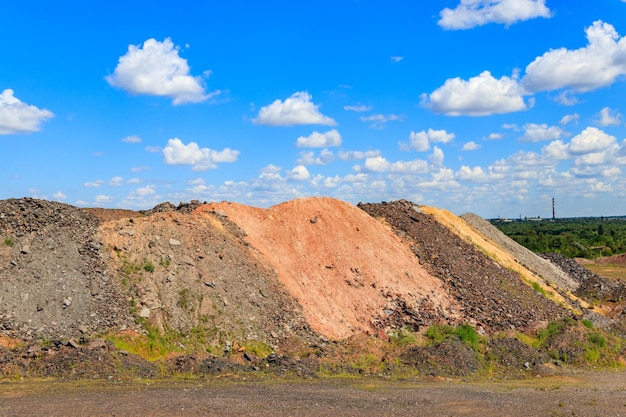This outdoor photo showcases a vivid, blue sky adorned with numerous puffy white clouds. Below the sky, the landscape features a diverse terrain with a flat dirt area leading up to a colorful hill composed of various types of dirt and clay. The hill exhibits distinct sections of gray, lighter gray, light clay, dark dirt, yellowish soil, and stone-colored areas. Among these mounds of dirt, there are scattered rocks and tufts of weeds sprouting from the ground. In the background, lush green trees and an indistinct building can be seen, partially obscured by foliage. A black tower rises among the greenery, adding vertical contrast to the landscape.